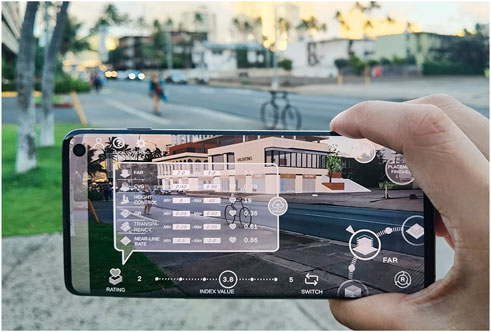A detailed and comprehensive caption combining all the inputs might look like this:

The image captures a bustling city street scene from a landscape perspective. In the immediate foreground, a Caucasian person's right hand is holding a smartphone horizontally. The phone screen, visible to the viewer, appears to be open to a camera application with various settings and menus displayed, including measurement tools and a "ratio" indicator. What’s on the phone screen mirrors the background, albeit with additional graphics and text.

In the mid-ground, the scene unfolds with a concrete sidewalk running horizontally to the left and right and extending forward into the distance. There is a bicycle parked near the edge of the sidewalk, and a person stands nearby, possibly looking to cross the street. On the left, a patch of green grass is dotted with two tall tree trunks, with more foliage visible further in the distance.

Across the street, a few low-rise buildings and houses are discernible, some appearing to be apartment structures. The background features taller palm trees hinting at a cityscape, possibly in California. The road is gray, and there are yellow traffic lines marking it. The entire scene is bright and detailed, reflecting a busy urban environment.